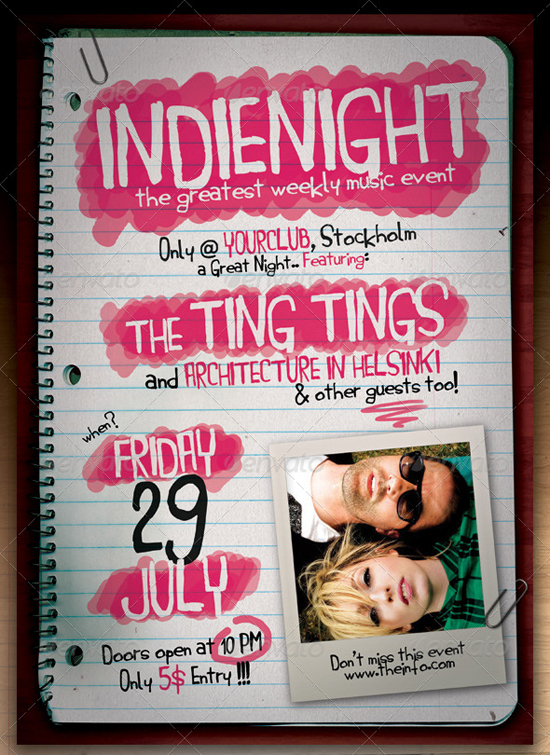In the image, we have a spiral notebook against a brown desk background. The notebook dominates the frame, with a paperclip holding some pages together on the upper left-hand corner. At the top in large white letters on a pink bubbly background, it reads "Indie Night," followed by "the greatest weekly music event" in smaller white letters. Just below this, against the lined notebook paper, it states "only at your club, Stockholm, a great night featuring the Ting Tings," with "The Ting Tings" again highlighted in large white all-cap letters. 

Below that, it mentions "and Architecture in Helsinki and other guests too." On the lower left-hand side, it states "Friday, 29 July," with "Friday" and "July" in all-cap white letters against pink backgrounds, and "doors open at 10 p.m." with 10 p.m. circled in pink. It also notes "only $5 entry," emphasized with three exclamation marks. 

In the bottom right-hand corner, there's a Polaroid picture of a man and woman. The man, wearing sunglasses and having short brown hair, lies beside a smiling woman with short blonde hair. She wears a green and black shirt, and her hair appears messy. The image is clipped to the notebook page and annotated with "don't miss this event, www.theinfo.com." The overall background of the image is bright pink, with the black and white lettering strikingly standing out.